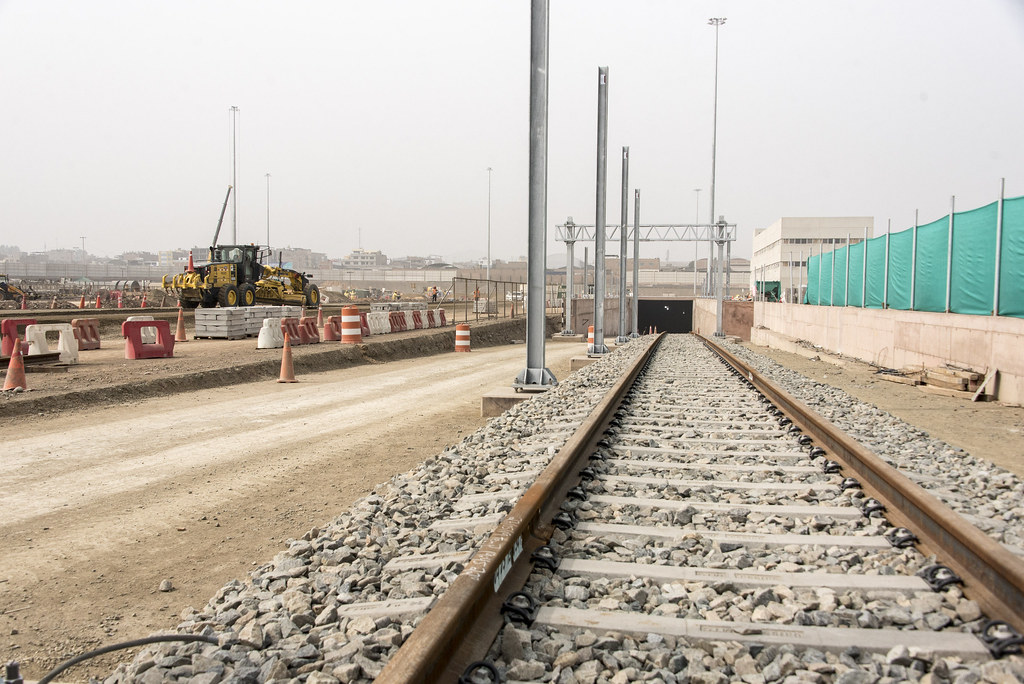The photograph, taken outdoors during the daytime, features a pair of rusted brown railroad tracks that seem to vanish into a distant tunnel, framed with gray gravel underneath. The tracks, reinforced with horizontal slats of white wood, extend from the bottom center and the right-hand corner of the rectangular frame, measuring approximately 6 inches wide by 4 inches high. To the left of the tracks lies a dirt drive, suggesting ongoing construction, as evidenced by orange cones and work barriers. A large yellow tractor or bulldozer is visible on this side, hinting at further development. Adjacent to the tracks on the right, several tall, gray metal columns stand upright, potentially part of an emerging platform structure. This side also features a stone wall topped with a green fence, and a white square building, all set against a backdrop of a foggy or smoggy sky. The overall scene is dominated by light brown and tan hues, complemented by light blue and gray tones in the distance. The combination of gravel, stone, and construction elements suggests an area in transformation, with signs of a town faintly visible in the hazy background.